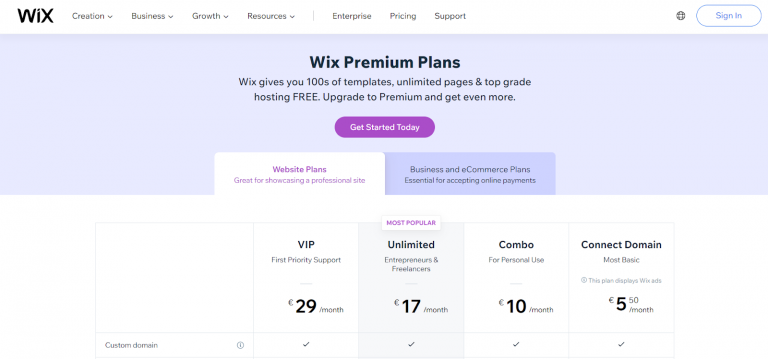The image showcases a webpage from Wix's official website, detailing its premium plans. The webpage is designed with a clean, white background and is horizontally oriented. At the top of the page, there are various pull-down menus labeled "Creation," "Business," "Growth," and "Resources." Additionally, there are clickable links for "Enterprise," "Pricing," and "Support." 

In the top right corner, there's a white oval-shaped button outlined in blue, labeled "Sign In." Below the main navigation bar, a lavender text banner displays the message "Wix Premium Plans," highlighting the benefits of Wix, such as access to hundreds of templates, unlimited pages, and top-grade hosting for free. The banner encourages users to upgrade to premium for more features.

Beneath this, a prominent purple oval button labeled "Get Started Today" is situated for users to begin the process. The page then details different premium plans in a text box: VIP for £29 a month, Unlimited for £17 a month, Combo for £10 a month, and Connect Domain for £5.50 a month. There are also clickable tabs for "Website Plans" and "Business & eCommerce Plans," providing further options for the user.